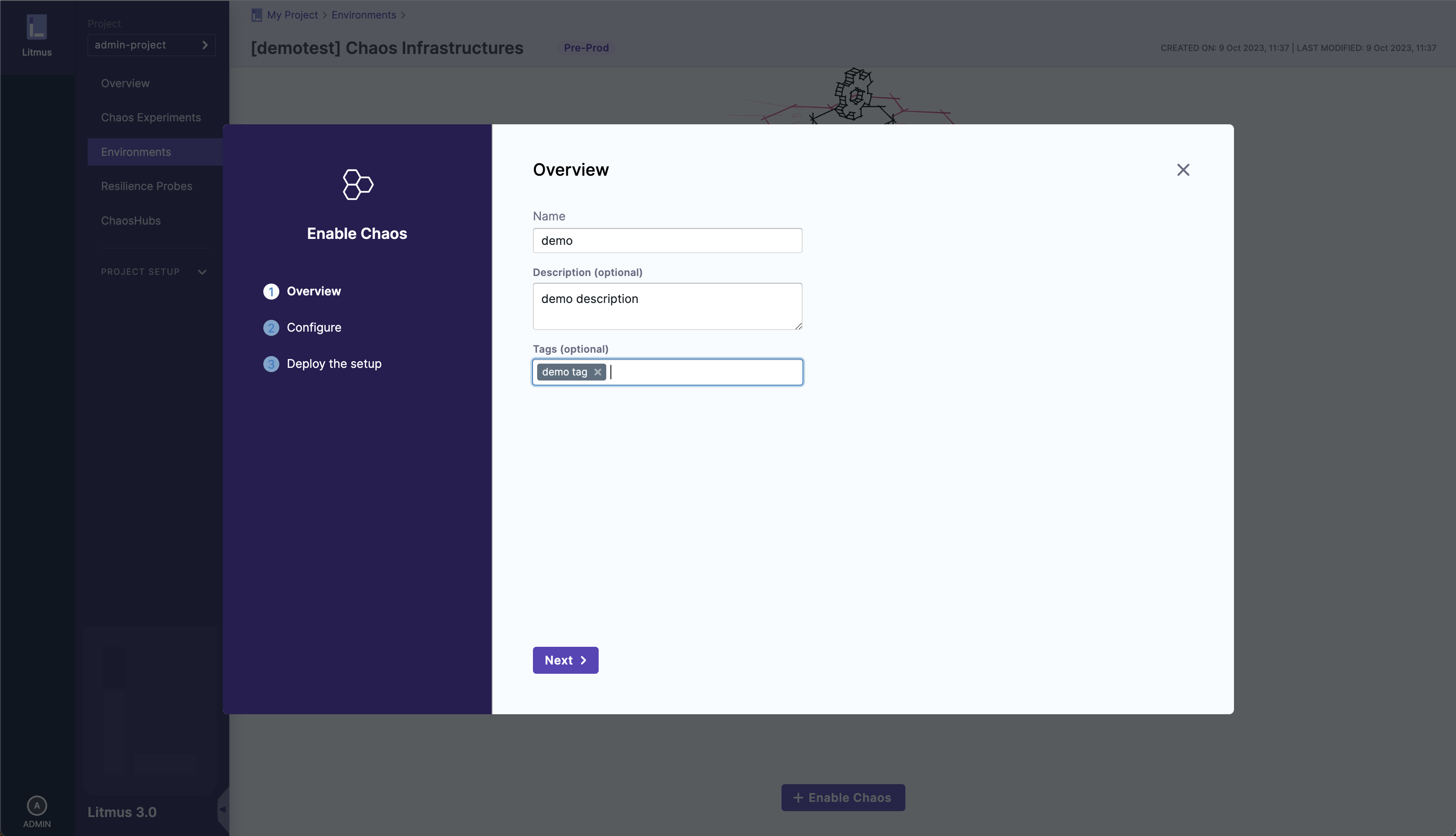The image depicts a two-layer interface primarily showcasing an 'Enable Chaos' screen with a honeycomb pattern consisting of three merged cells. The interface is divided into three sections: "Overview," "Configure," and "Deploy Setup," with the current view focusing on the "Overview" section. Here, users are prompted to enter a name, description, and tags for their setup, with "Demo" pre-filled as the default name. The interface also includes a 'Next' button to proceed to the "Configure" step. In the background, there is a faint, hard-to-read page that appears to be related to an online marketplace or network, though details are unclear. A navigation panel is visible on the left, albeit with illegible text, while on the right, the interface displays "Demo Test Chaos Infrastructures" and a prominent "Enable Chaos" button, which the user previously clicked to reach this screen.